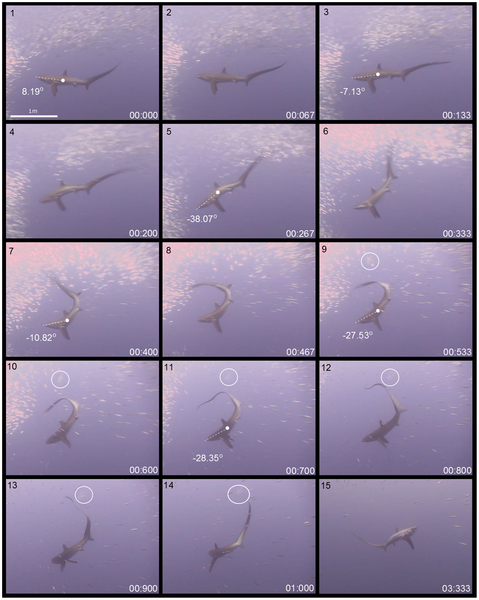This rectangular image, bordered in black, is subdivided into 15 smaller frames arranged in a grid of five rows by three columns, each separated by vertical and horizontal black lines. Each frame captures a different moment of a shark swimming through the water, viewed from above. In the upper left corner of each frame, a black number from 1 to 15 labels the sequence. In the lower right corner, a white timer starts at 0 seconds in the first frame and progresses to 3.333 seconds in the last frame. 

The scene is bathed in shades of bluish-white, showcasing the shark's progression through the water. Initially, the shark begins at 0 seconds and -8.19 degrees in frame one. As the sequence continues, the timer advances while the shark exhibits different swimming motions, such as diving and rising. Notably, the shark's tail curves and extends distinctly in several frames, reflecting its dynamic movements. By the final frame, the shark has ascended and some fish can be seen surrounding it.